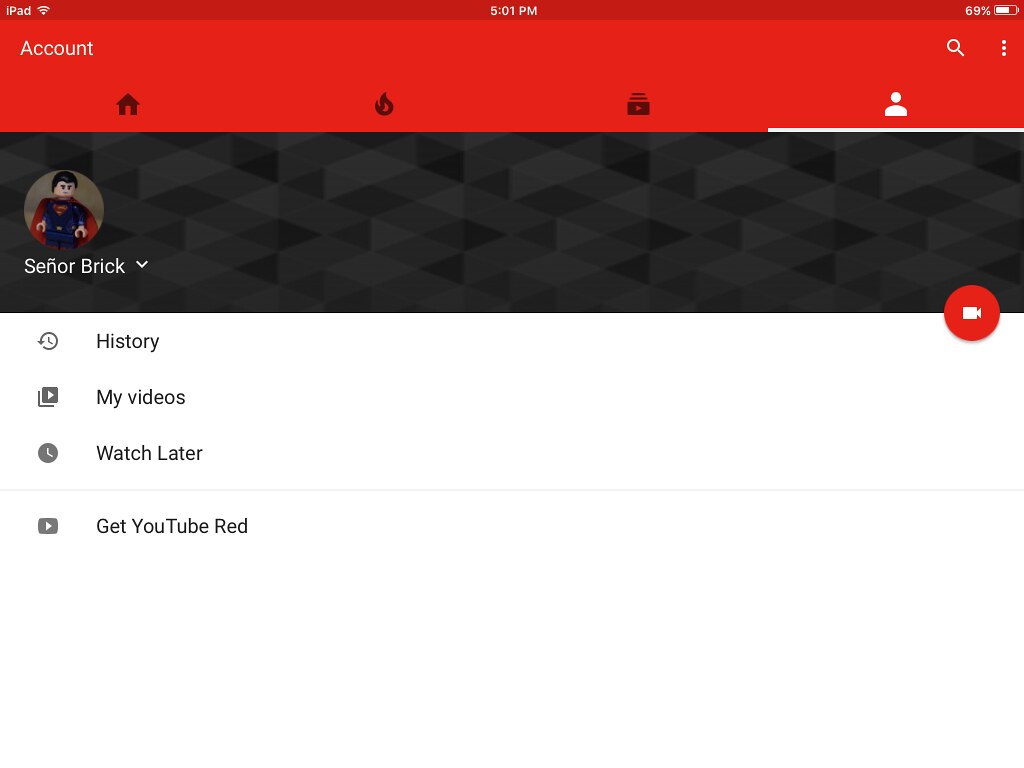This is a detailed description of a screenshot from an iPad. The top of the screen features the status bar, displaying "iPad" in white font on the left, "5:01 PM" in the center, and the battery level at 69% on the right. Below the "iPad" label, the word "Account" is also displayed in white font.

The background beneath this status bar is red and patterned with various icons. The row of icons includes a black house icon, a black flame-like icon, a black play button resembling the YouTube symbol, and a black icon that looks like a file folder with an arrow in the center. There is also a white icon depicting a person's head and shoulders.

Lower on the screen, there is a user's profile picture set against a black, geometric background. The profile image features the Superman character, dressed in his classic blue outfit and red cape, with the iconic "S" emblem on his chest and black hair. Below the image, the username "Senor Brick" is written in white font.

On the opposite side of the profile picture, there is a red camera icon. The area below this section features a list of labels against a white background, with corresponding icons in black font:
- "History" next to a clock icon
- "My videos" next to a square icon with a play button
- "Watch later" next to a clock-looking icon
- "Get YouTube Red" next to a square icon with an arrow in it

This setup suggests that the screenshot depicts the account section of a YouTube interface, displaying various navigation options and the user's profile information.